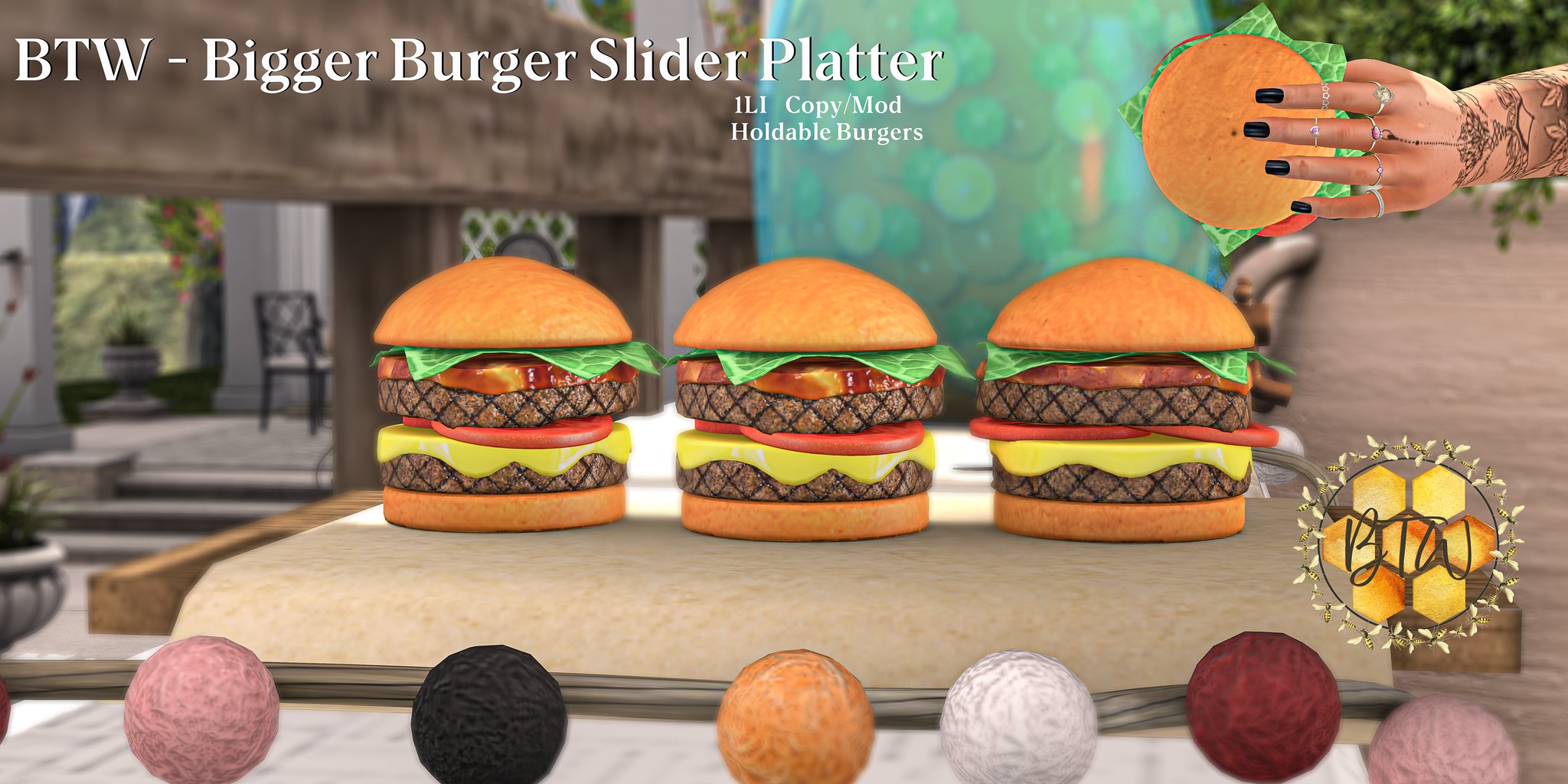This digital illustration showcases a trio of meticulously detailed, cartoonish or AI-generated hamburgers placed side-by-side on a tan-colored surface. Each burger is crafted with a top brown bun, crisp green lettuce, vibrant red tomatoes, a juicy grilled patty, more tomatoes, melted yellow cheese, a second patty, and a bottom bun. In the background, elements of a cozy patio setting are visible, including a wooden beam, chairs, plants, and a lattice structure. A large blue orb shape sits behind the burgers, adding a touch of surrealism. On the right side, a left hand emerges, adorned with black painted fingernails, several rings, and tattoos, holding one of the burgers aloft. The top left of the image features bold text: "BTW Bigger Burger Slider Platter," with smaller white text below reading "ILI copy mod holdable burgers." The bottom of the image displays a series of colored circles—pink, black, tan, white, maroon, and another pink—and a logo for BTW, encircled by bumblebees around a honeycomb hive.